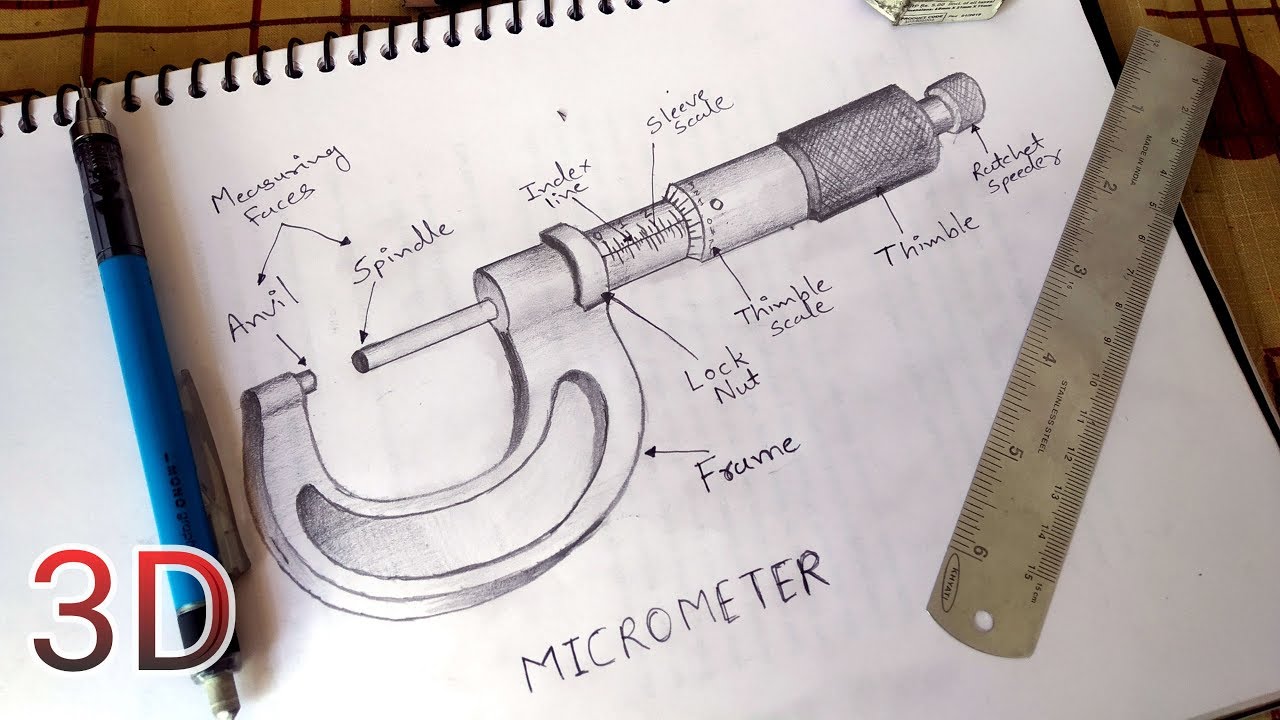The image is a rectangular, horizontal photograph showcasing a top view of a spiral-bound drawing book placed on a gray or brown surface. On the open page of the drawing book, there is a detailed sketch of a micrometer, drawn in black and gray. Various parts of the micrometer are meticulously labeled, including the spindle, anvil, lock nut, ratchet, thimble, thimble scale, sleeve scale, index line, the U-shaped frame, and measuring faces. The sketch is executed on plain white paper within the notebook, with "micrometer" handwritten in large capital letters near the sketch. To the left of the notebook, a blue clicker pen with a black bottom rests on top of the book, partially overlaid by the letters "3D" in the lower left corner of the image. The "3D" text is primarily red with the top parts outlined in white and the bottom halves in gray. To the right side of the drawing book, a gray six-inch metal ruler is placed at an angle, extending diagonally from the lower left towards the upper right, across the notebook.